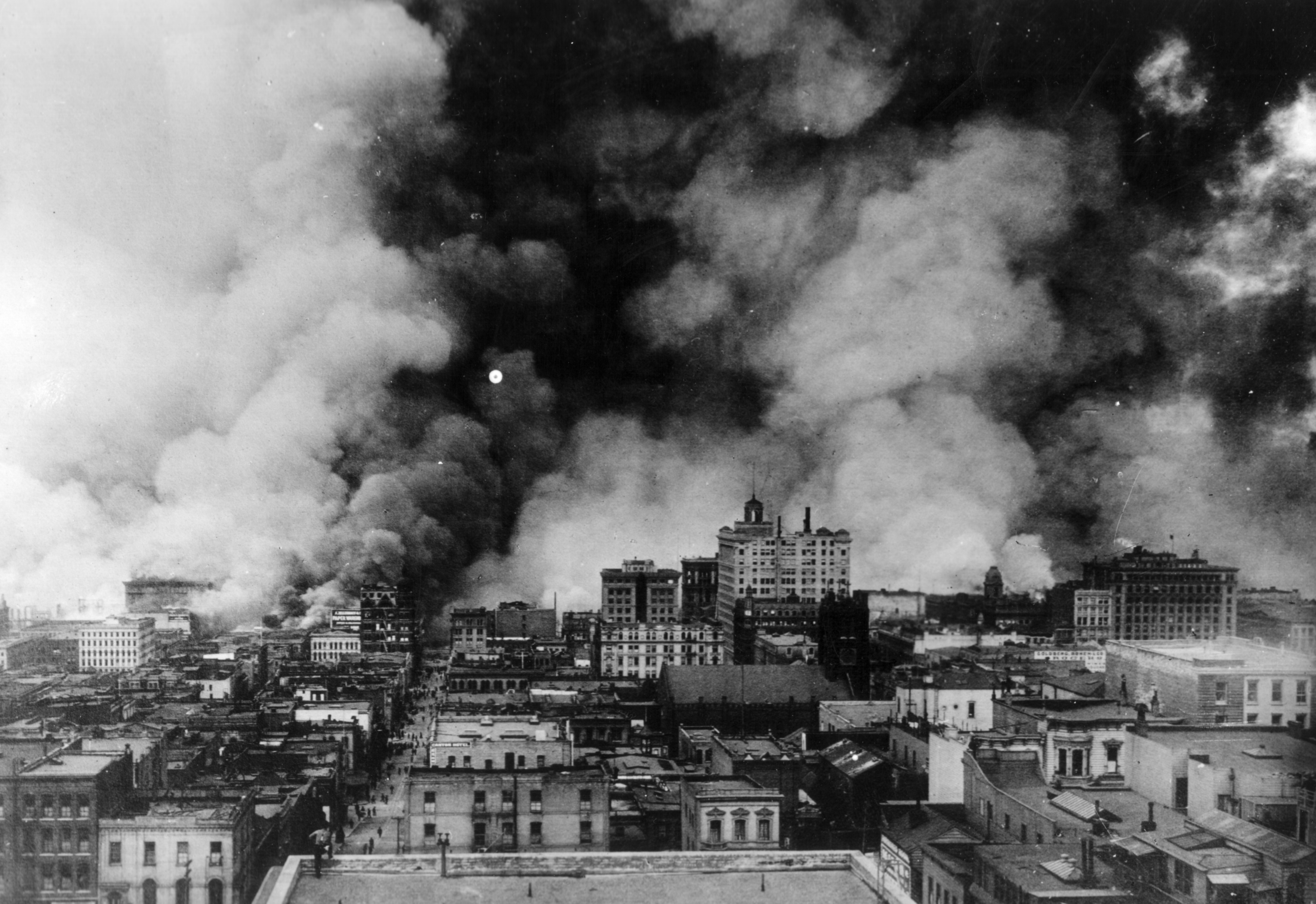This historic black and white photograph captures a densely populated city engulfed in smoke. The image prominently features a variety of buildings ranging from three to ten stories high, with many displaying numerous windows. The foreground reveals a city street bordered by unique, albeit somewhat dirty, edifices. Towards the left, a road stretches into the distance, while clusters of buildings dominate the midsection and right side of the image. The scene contains mostly rectangular, boxy structures, some of which have visibly dark, perhaps damaged, rooftops.

In the background, a dramatic scene unfolds: billowing black, gray, and white smoke rises ominously from the buildings, suggesting a massive fire consuming the skyline. The entirety of the sky is obscured by this thick smoke, creating a chaotic and almost apocalyptic atmosphere. Although the specific location remains uncertain, the image vividly portrays a moment of urban crisis, accentuated by the stark contrast between the towering structures and the overwhelming presence of smoke.